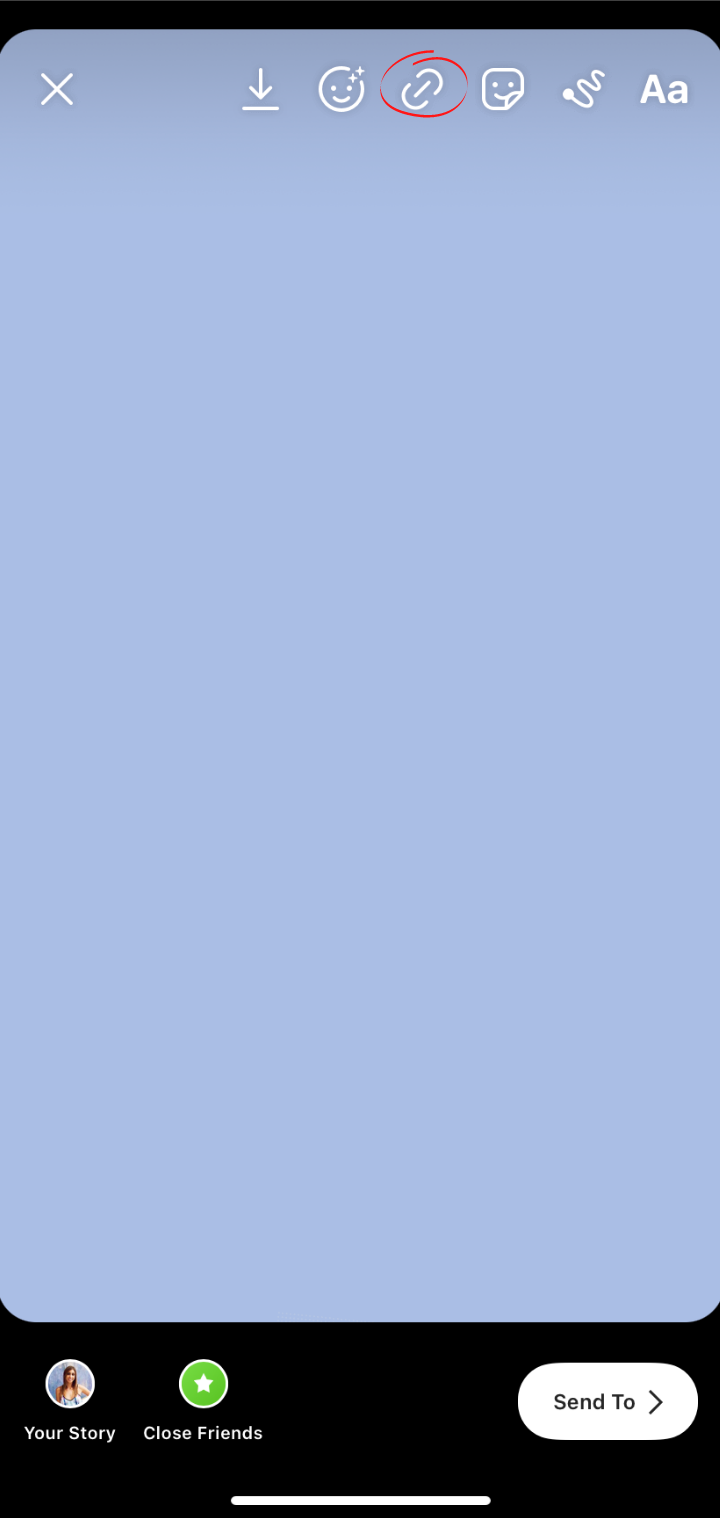This image showcases the user interface of a social media app, likely Instagram, during the story creation process. At the top of the screen, from left to right, there are multiple icons: 

1. An **exit button** to close the story creation screen without saving.
2. A **download button**, represented by a downward arrow, which saves the current story to the device.
3. An **effects button**, depicted with sparkles, that allows users to add filters or effects to their story.
4. A **link button**, illustrated as a chain link, enabling users to add a link to the story so viewers can swipe up to visit a website.
5. A **stickers button**, shown as a smiley face within a square, which lets users add stickers, GIFs, polls, or other interactive elements.
6. A **draw button**, represented by a wavy line, to draw or doodle on the story using varying colors and brush sizes.
7. A **text button**, marked by “AA”, to add text to the story with various font options and styles.

The main screen currently displays a plain blue background, acting as a placeholder or default screen. At the bottom, there are buttons labeled "Your Story," "Close Friends," and "Send To," providing options for sharing the customized story. This user interface enables users to personalize and enhance their stories with a wide array of interactive elements, ensuring a creative and engaging social media experience.